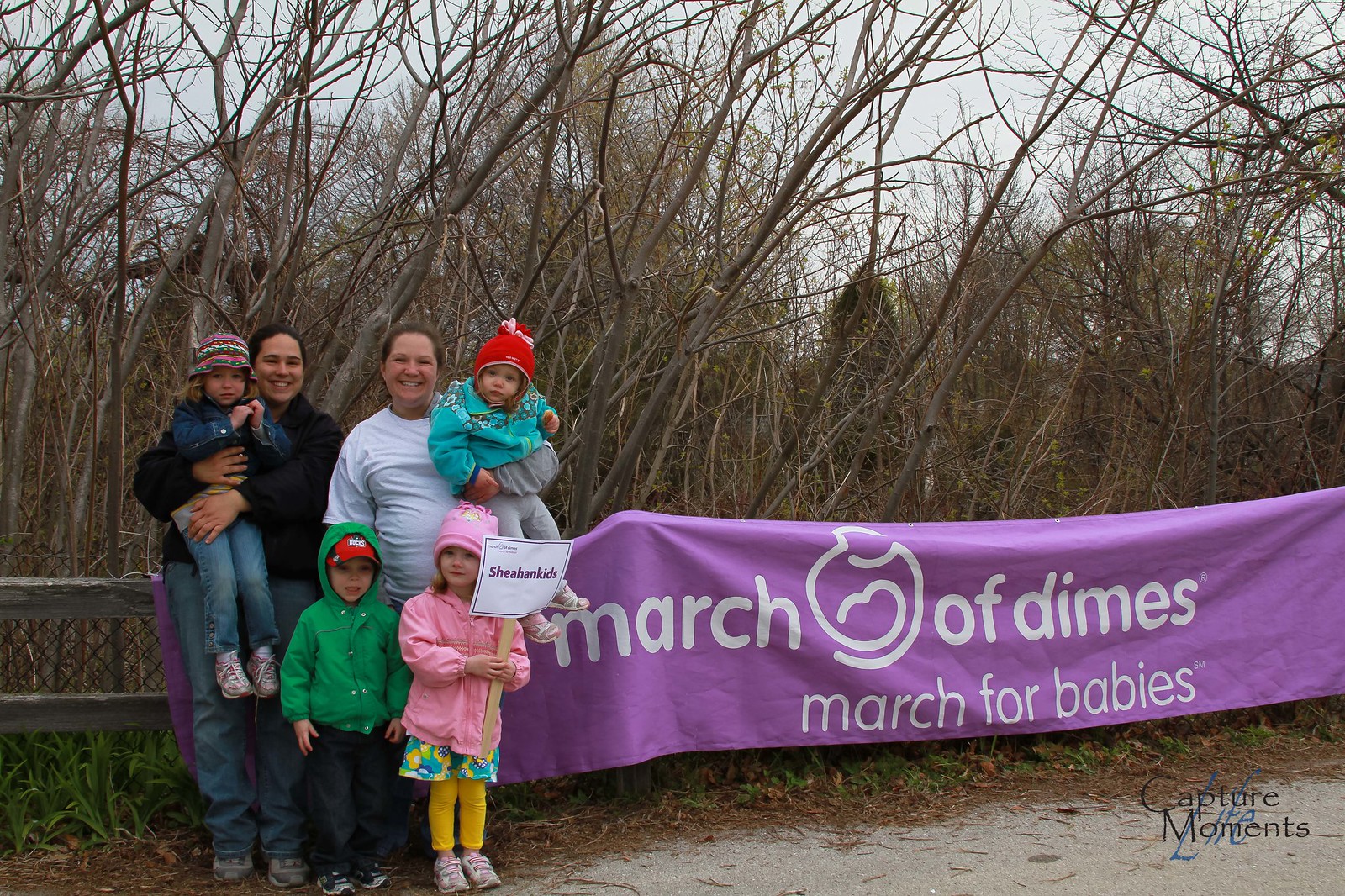In this outdoor photograph, two families stand together in front of a purple banner that reads "March of Dimes, March for Babies," attached to a wooden fence. The scene unfolds on a road bordered by green grass with a backdrop of leafless trees, indicating a fall setting under an overcast sky. On the left, a woman in a black sweatshirt and blue jeans cradles a young girl dressed in all denim. Both are smiling warmly at the camera. To their right, another smiling woman, chubby and wearing a white t-shirt, holds a little girl, possibly four or five years old. In front of this woman stand two more children: a young boy in a green jacket on the left and a young girl in a pink jacket on the right. Among them, the young girl holds a sign that reads "SHEHANDKIDS." The group exudes a sense of unity and joy as they participate in the event, capturing a cherished family moment.